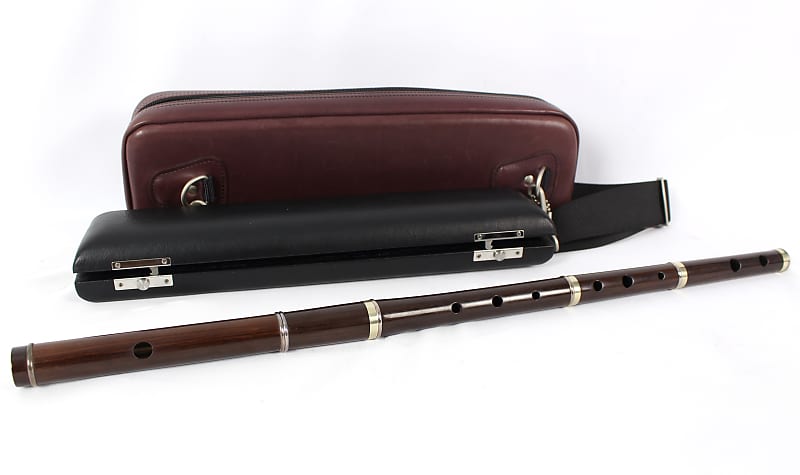The photograph showcases a detailed image of a musical instrument reminiscent of a flute or refined recorder, featuring a primarily brown body that appears to be either wooden or brown plastic, adorned with silver rings. The flute-like instrument, which likely disassembles at the silver bands for storage, is displayed prominently against a white background, suggesting it was taken in a lightbox or the background was digitally removed.

In the background, there are two cases: a black hardback case with chrome hinges and clasps that probably securely holds the flute, and a larger, burgundy case with a zipper at the top and a black strap, presumably designed to carry the hardback case and additional accessories. The black case is positioned slightly open or ajar, showing its silver clasps, while the burgundy case appears to be a secondary, larger carrying option, possibly made from leather or vinyl.